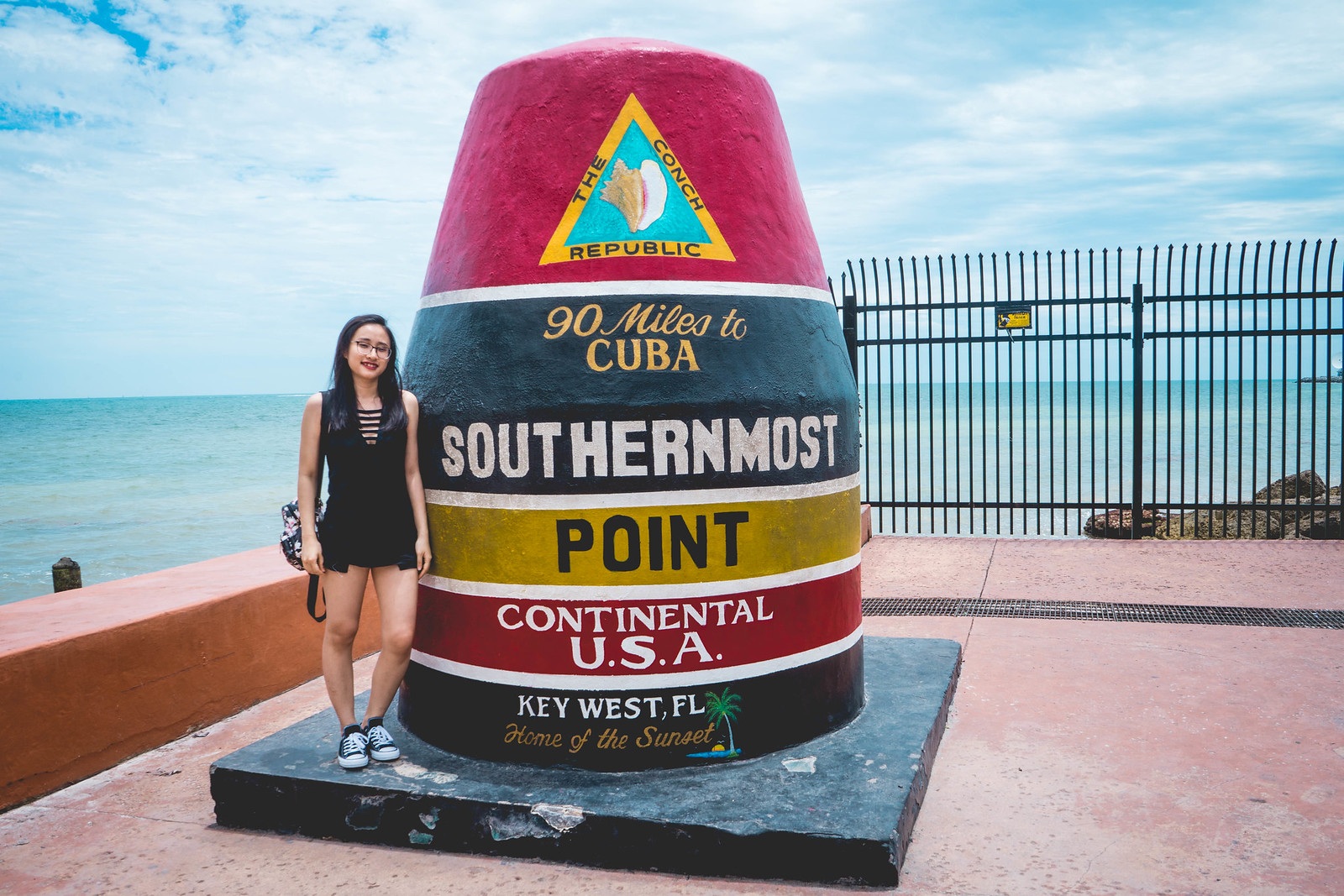A young girl, dressed in a black outfit with a purse on her right arm, stands next to the iconic Southernmost Point buoy in Key West, Florida. The buoy, which appears almost statue-like and is roughly eight to nine feet tall, boasts vibrant colors and distinct markings. The very top is cone-shaped and painted red with a yellow-bordered triangle bearing the label "The Conch Republic" and a conch shell illustration. Below this, on a black background, the text "90 miles to Cuba" is inscribed in gold. Further down, in white letters on a black circular background, it reads "Southernmost," followed by "Point" in black on a gold background. The lower section of the buoy features the text "Continental USA" in white against a red backdrop, and finally, at the bottom, "Key West, Florida, home of the sunset" is written in white on a black background, accompanied by a small illustration of a palm tree.

The girl, with dark black hair flowing over her front, wears black low-top sneakers and stands smiling on the buoy's black base. The scene is set against a picturesque backdrop of white clouds dotting a blue sky, with the blue waters of the Gulf stretching out behind her. The buoy stands on a red granite structure with a slight border to the left and a metal fence in the background, marking this famous tourist site.